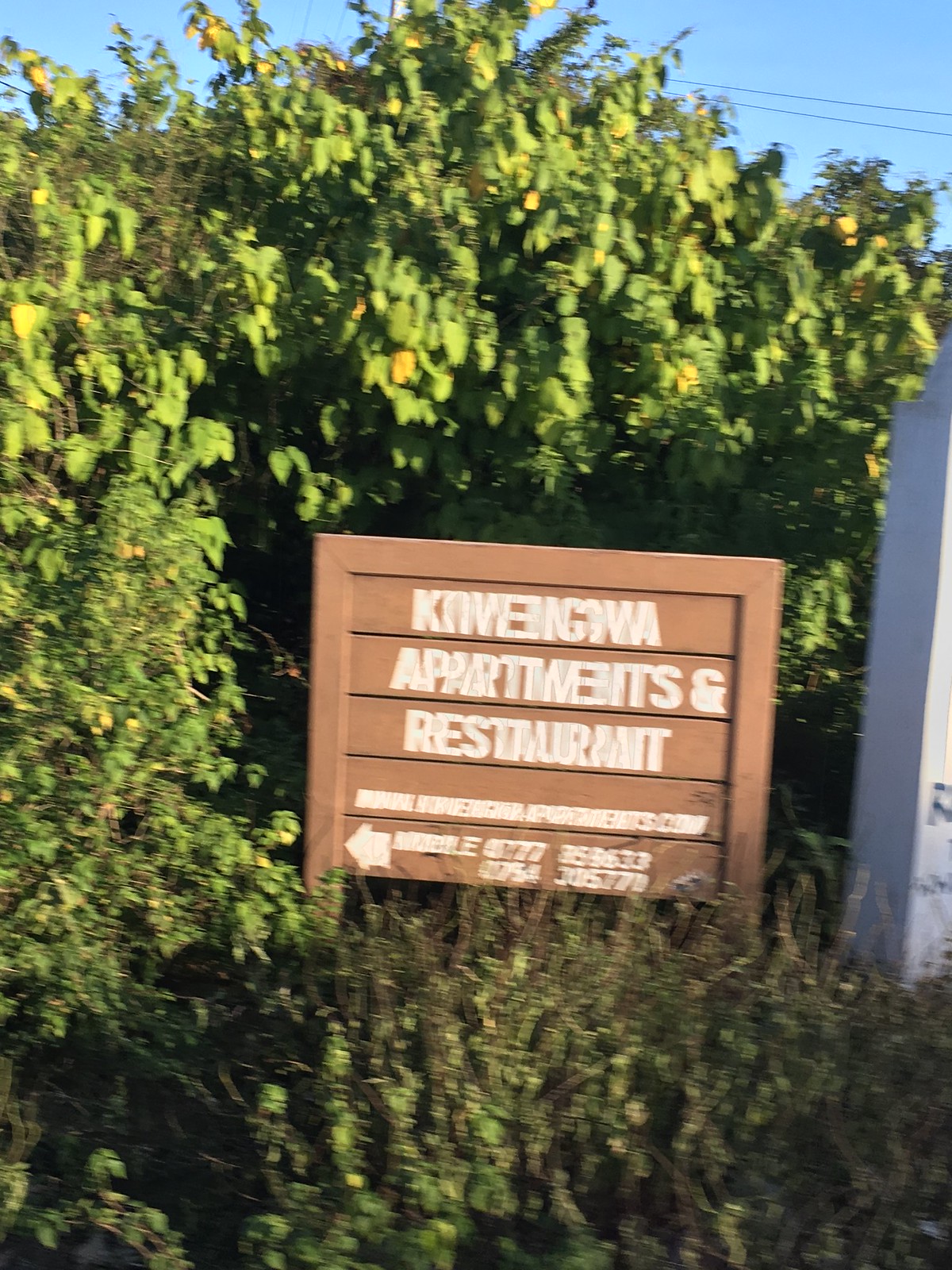This color photograph, captured in portrait mode during daytime, showcases a well-maintained outdoor setting. The background is densely filled with large, vibrant green bushes, interspersed with a few yellowing leaves, adding a touch of autumnal hue. Prominently featured in the scene is a rustic wooden sign, framed in brown wood with horizontal planks filling the square shape. 

Although the text at the top of the sign is blurred and overlapping, rendering it partially illegible, it appears to be AI-generated. The word "apartments" is discernible, followed by "restaurant." Additional text and numbers are present, but their clarity is compromised by the overlapping script. An arrow pointing to the left is also visible on the sign, suggesting directions to the named locations.